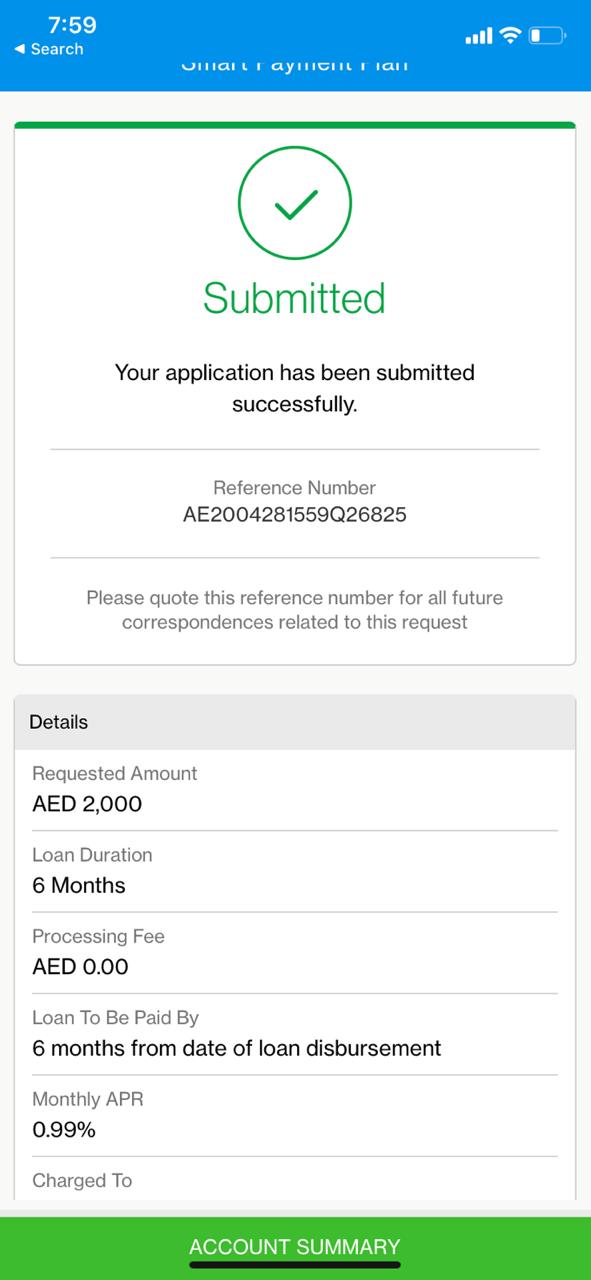A mobile phone screenshot, taken at 7:59, shows a payment application (partial text visible: "Smart Payment..."). Despite full signal strength, the battery is notably low. The screen highlights a completed application process with a prominent check mark and the message: "Submitted. Your application has been submitted successfully." Below, a long reference number is provided with instructions to quote it for all future correspondences related to the request. The application details include:

- Requested amount: AED 2000
- Loan duration: 6 months
- Processing fee: AED 0.00
- Loan to be paid by: 6 months from the date of loan disbursement
- Monthly APR: 0.99%

Further down, a "Charged To" section is partially visible, but the specifics are not displayed due to the screen not scrolling down completely. At the footer, a green box labeled "Account Summary" suggests the current page or a navigation option. This screenshot details the successful submission of a loan application and its relevant terms.